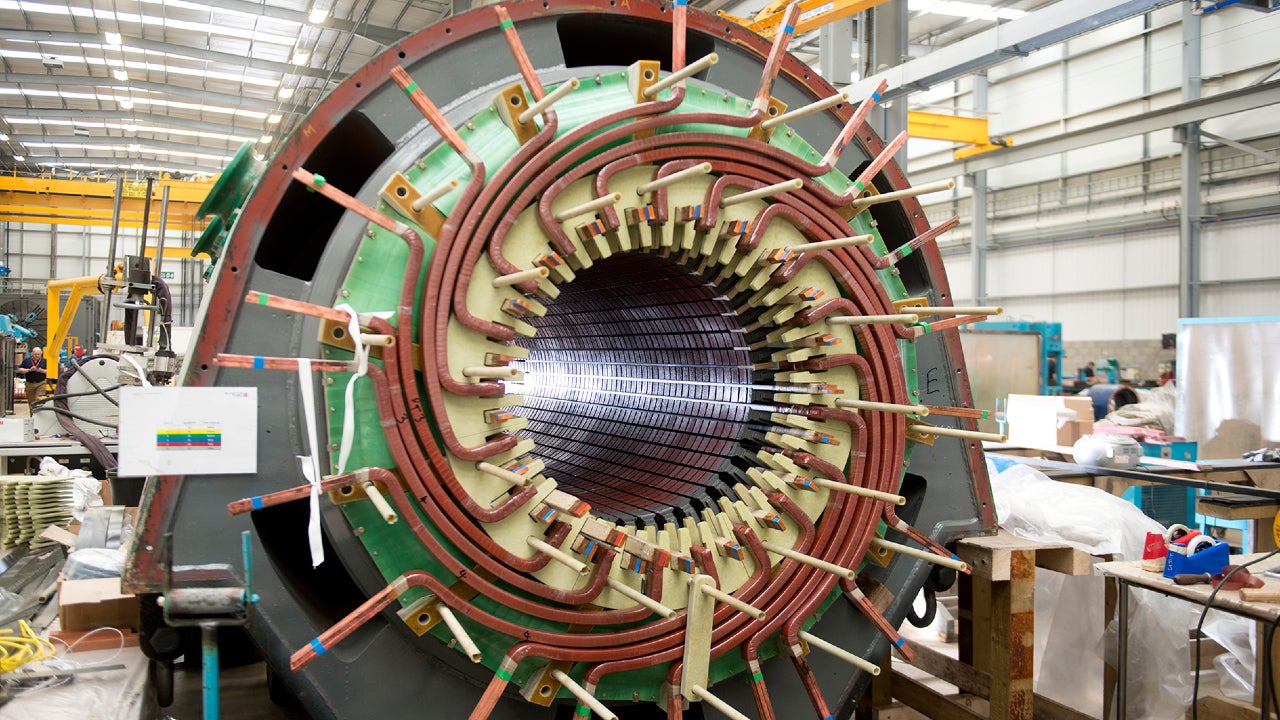Inside a bustling warehouse adorned with steel beams and cranes, a mysterious machine commands attention at its center. This large, cylindrical device, reminiscent of a brushless motor or an MRI tube stripped of its casing, reveals intricate inner workings. Copper coils intertwine with wires of various colors, predominantly tan, green, yellow, brown, orange, and pink, all converging into a complex network. The inner tube showcases shades of red and silver, while the exterior features a yellow circular structure from which the colorful wire tubes emerge, connecting to a formidable red metal arch. Surrounding the machine, the chaotic warehouse scene includes overhead lighting, a yellow bridge, scattered bars, and draped cloths. Nearby, a table holds tape holders, various wires, rollers, and a stack of papers or trays. The entire setting reflects a place of intense industrial activity, illuminated by sunlight that reflects off the intricate coils, with a chart adding to the enigmatic atmosphere.